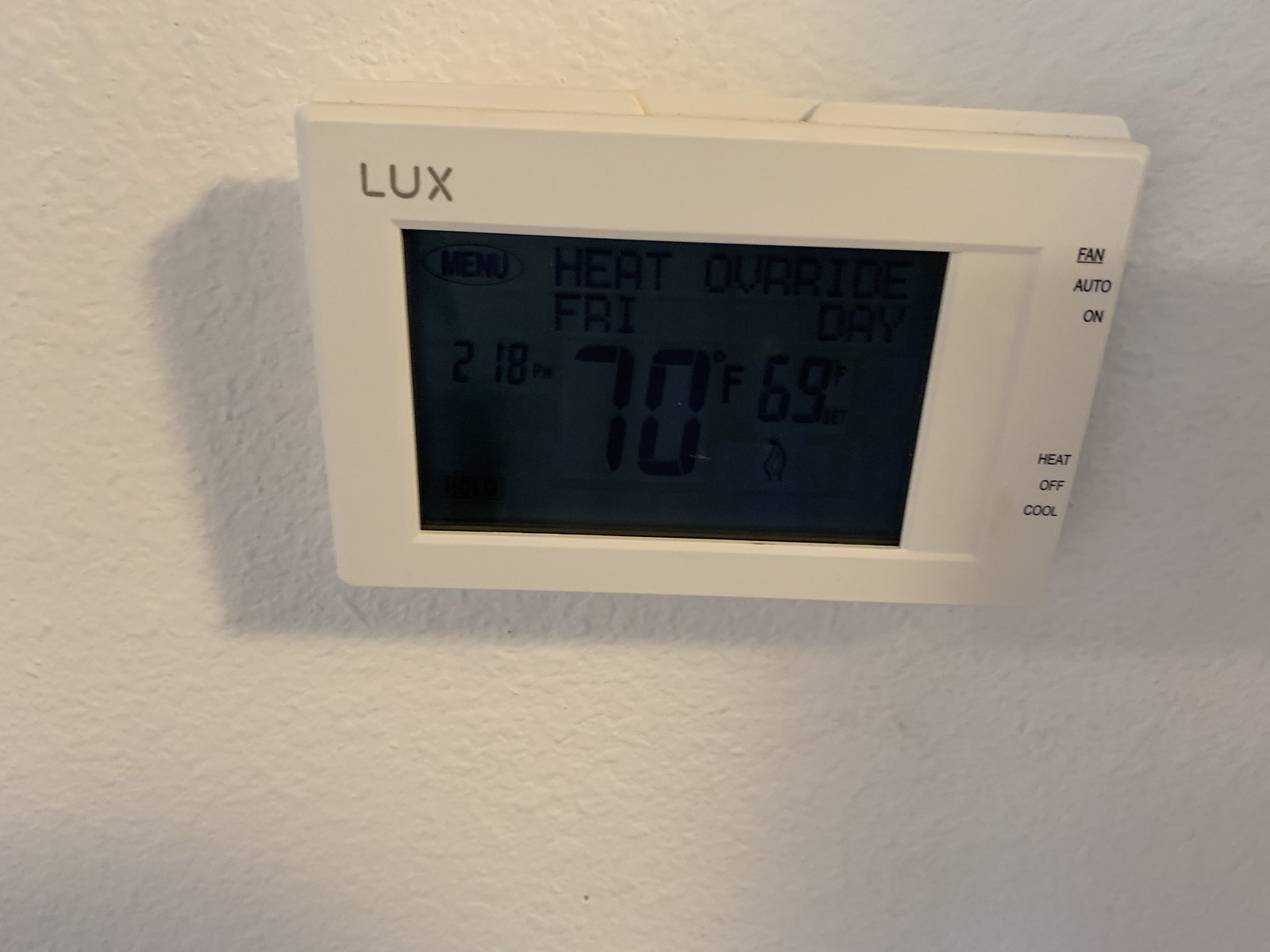This color photograph captures a rectangular thermostat mounted on a textured wall. The thermostat features a clean white border and prominently displays the brand name "LUX" in silver capital letters at the top. On the right-hand side of the device, you can see labels for Fan settings, including "Auto" and "On," as well as modes for "Heat," "Off," and "Cool," all written in bold black capital letters.

The central display of the thermostat is rectangular with a smoked glass appearance, featuring slightly faded information indicating a temperature of 70 degrees Fahrenheit, the current mode as "Heat," and the status "On." Additionally, it displays the day as "Friday."

The top of the thermostat includes a bezel with a distinctive design that is divided into two parts along the width, featuring angled indentations. The device appears slightly detached from the wall and is tilted downward at the right-hand corner, adding a sense of depth to the photograph.